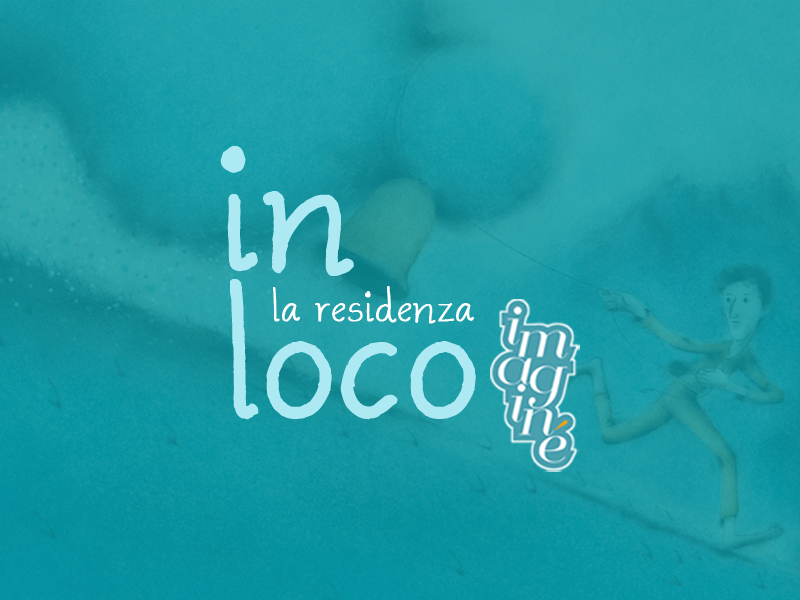The image features a textured, primarily light blue background with a cartoon-style character running in the bottom right corner. The character is a lanky male in an orange jumpsuit, tugging at a string attached to a floating bell. Superimposed over this scene, in the center of the image, is text in a playful, cartoony font. The main text reads "In Loco" with "La Residenza" running horizontally through the letters "OCO." Additionally, beneath this, the word "Imagine" is arranged in three lines, with the last letter "E" dropping vertically. The overall composition conveys an old-school cartoon vibe with a soothing teal, gray, white, and orange color palette.